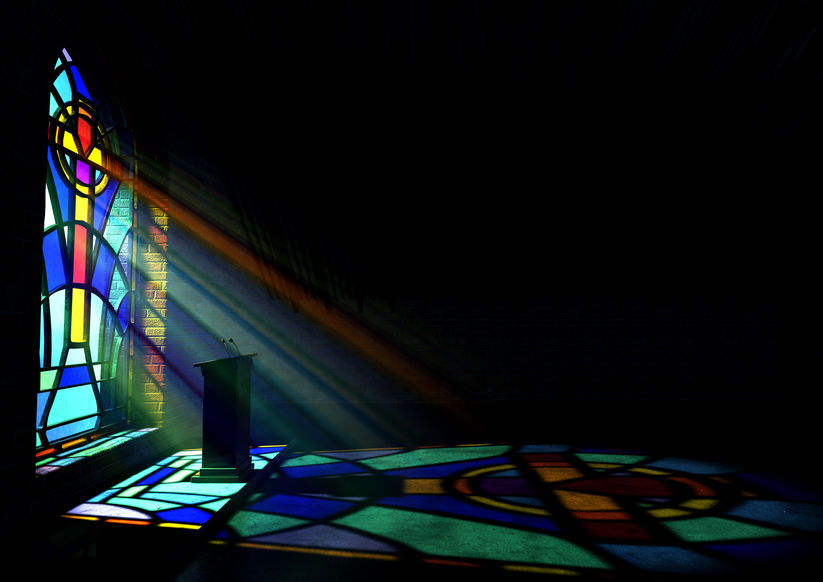This photograph captures a striking image of a darkened room, likely a church, illuminated solely by light streaming through a stained glass window. The stained glass, depicting a crucifix, projects an enlarged, colorful version of its intricate design onto the floor below. The primary colors in the stained glass are red, yellow, and blue, accented with green and orange. These hues spread across the room in vibrant rays, creating a vivid contrast against the dark surroundings. Situated before the window stands a podium with a microphone, framed by a backdrop of partially visible brick walls. The window, reaching up to a point and surrounded by brick, casts colorful beams that reveal the intricate design and the ambient beauty of the scene.